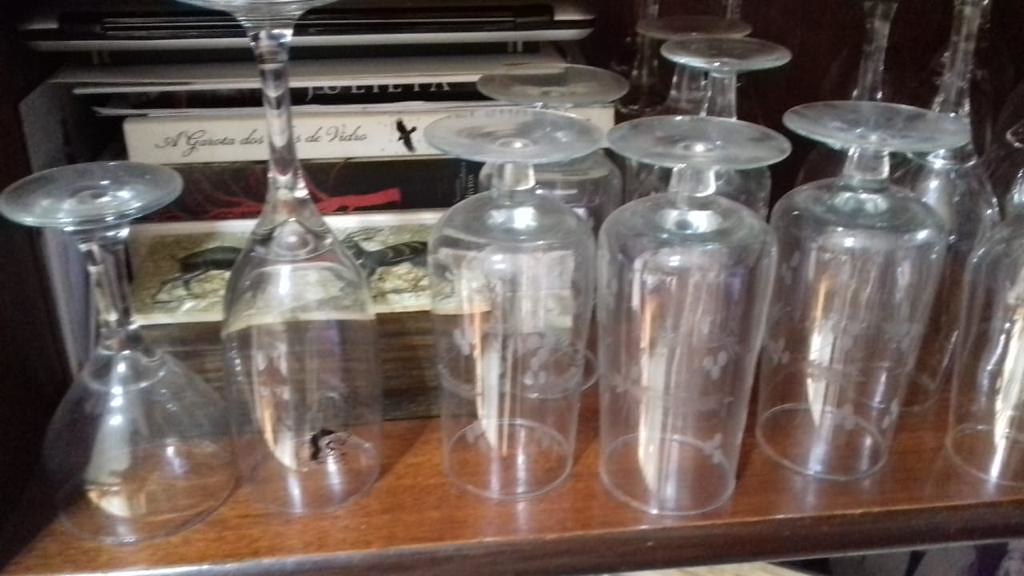The image showcases a collection of various glasses meticulously arranged on a wooden countertop. The glasses, numbering around twelve though partially cut off, exhibit a range of types including wine glasses, whiskey decanter glasses, and port glasses. Some of the glasses are uniquely designed with intricate etchings, possibly floral, and all are turned upside down, suggesting they might have been recently cleaned or are being displayed. The scene is slightly out of focus, imparting a vintage or antique quality to the photograph. Behind the glasses, there is a bookshelf or a stack of books with varied covers, including black and white, black and red, and one featuring an image that could be deer. The overall atmosphere hints at an antique shop or a cozy home setting, adding a touch of nostalgia to the image.